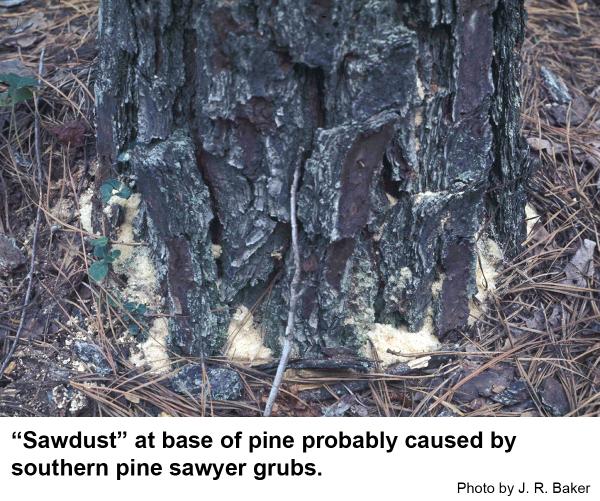This close-up image captures the base of a large pine tree, featuring dark, almost black, bumpy bark with hints of gray, and patches of purple and white. At the tree's base, there is a scattering of light tan sawdust, likely caused by southern pine sawyer grubs. Surrounding the tree are dry pine needles, dead vegetation, a few small leafy green plants, and some twigs, evoking a late-season, possibly autumnal, atmosphere. The text "sawdust at base of pine, probably caused by southern pine sawyer grubs" is displayed in black font at the bottom of the image, with "photo by J.R. Baker" in smaller text at the bottom right.